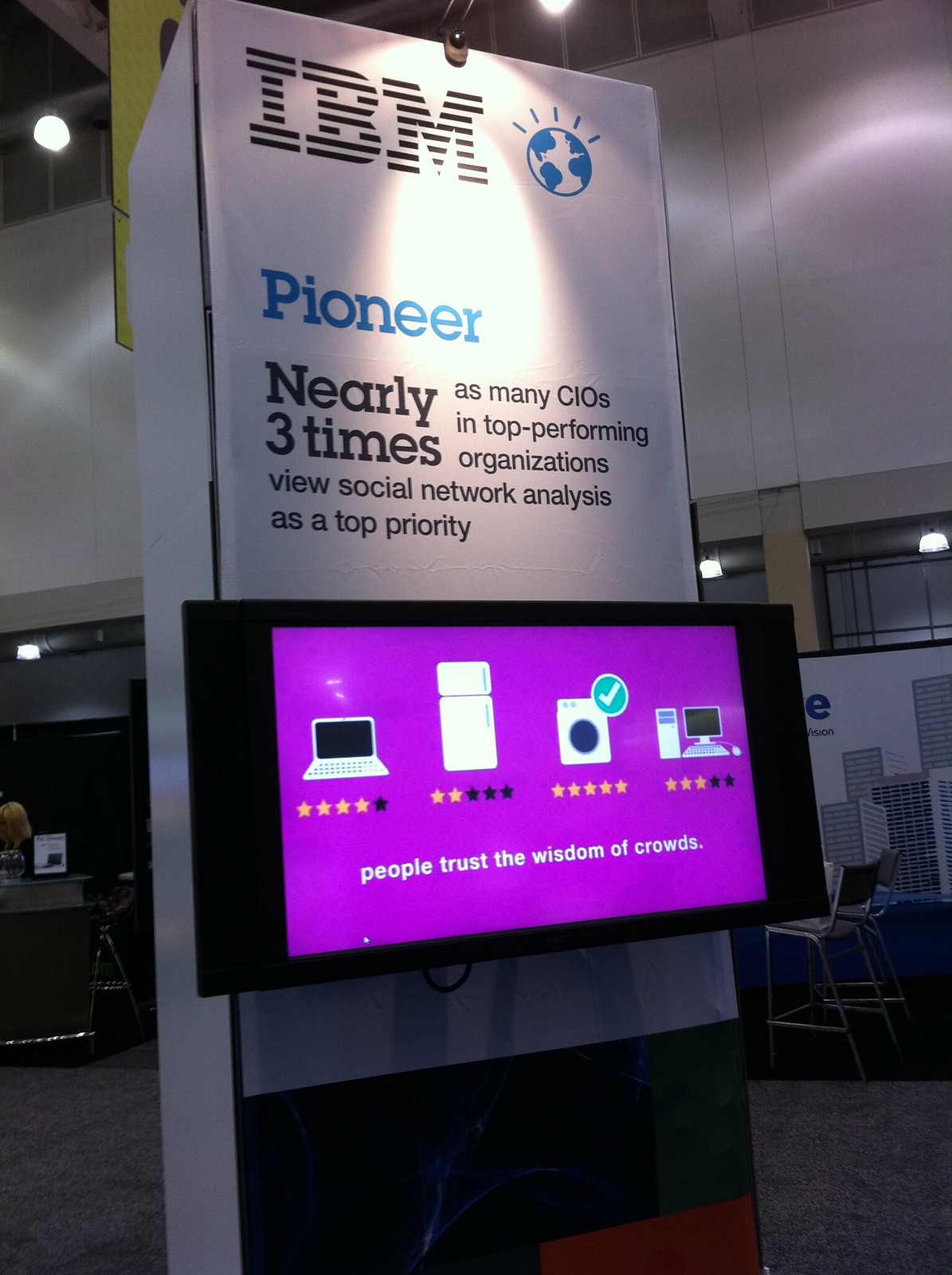The image features an indoor kiosk in a dimly-lit area with high ceilings and overhead lights, surrounded by white and gray walls. The focal point of the ad is a white vertical sign featuring the IBM logo at the top with a blue globe and horizontal lines. Below the logo, the word "Pioneer" is prominently displayed, followed by text in black that reads, "Nearly three times as many CIOs and top-performing organizations view social network analysis as a top priority."

Attached to the sign is a large, black monitor with a purple screen. The screen displays several objects with rating indicators: a white laptop with four out of five gold stars, a refrigerator with two out of five gold stars, a front-loading washing machine with a green check mark and five gold stars, and a white desktop computer and tower with three out of five gold stars. The screen also carries the text in white letters, "People trust the wisdom of crowds."

Beneath the purple screen, the sign transitions into a white bar and a dark blue bar. The scene around the kiosk includes various office-like elements such as gray desks, chairs, and other signs in the vicinity, contributing to the professional ambiance of the area.